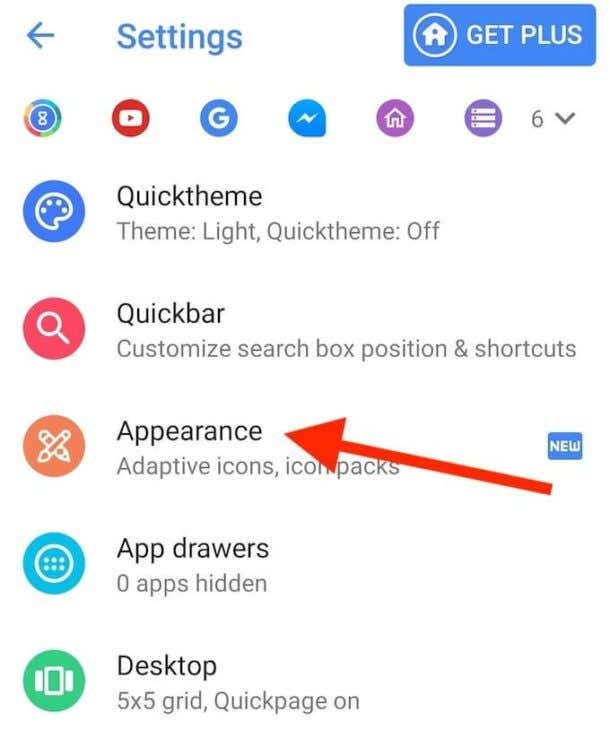The image depicts a settings page with various configuration options. At the top left, an arrow allows users to navigate back to the previous page. In the upper right corner, there's a blue button featuring "Get Plus" in white text, alongside a circular icon with a simplistic white house illustration, symbolizing the home button.

Below this section, the interface displays a series of icons corresponding to different applications, including a "G" for Google, a YouTube icon, a possible Twitter icon, and another home symbol in purple. The following options are listed under various headings:

- **Quick Theme**: Options include "Theme Light" and "Quick Theme Off."
- **Quick Bar**: Allows customization of the search bar's position and shortcuts.
- **Appearance**: Highlighted by a prominent red arrow and a blue "New" label, indicating this is a new or important section. Options here include "Adaptive Icons" and "Icon Packs."
- **App Drawers**: Indicates that "0 Apps Hidden."
- **Desktop**: Displays settings like a "5x5 grid" and "Quick Page On."

The significant red arrow pointing to the "Appearance" section suggests it is a focal point for the user, either as a new feature or an important customization option.